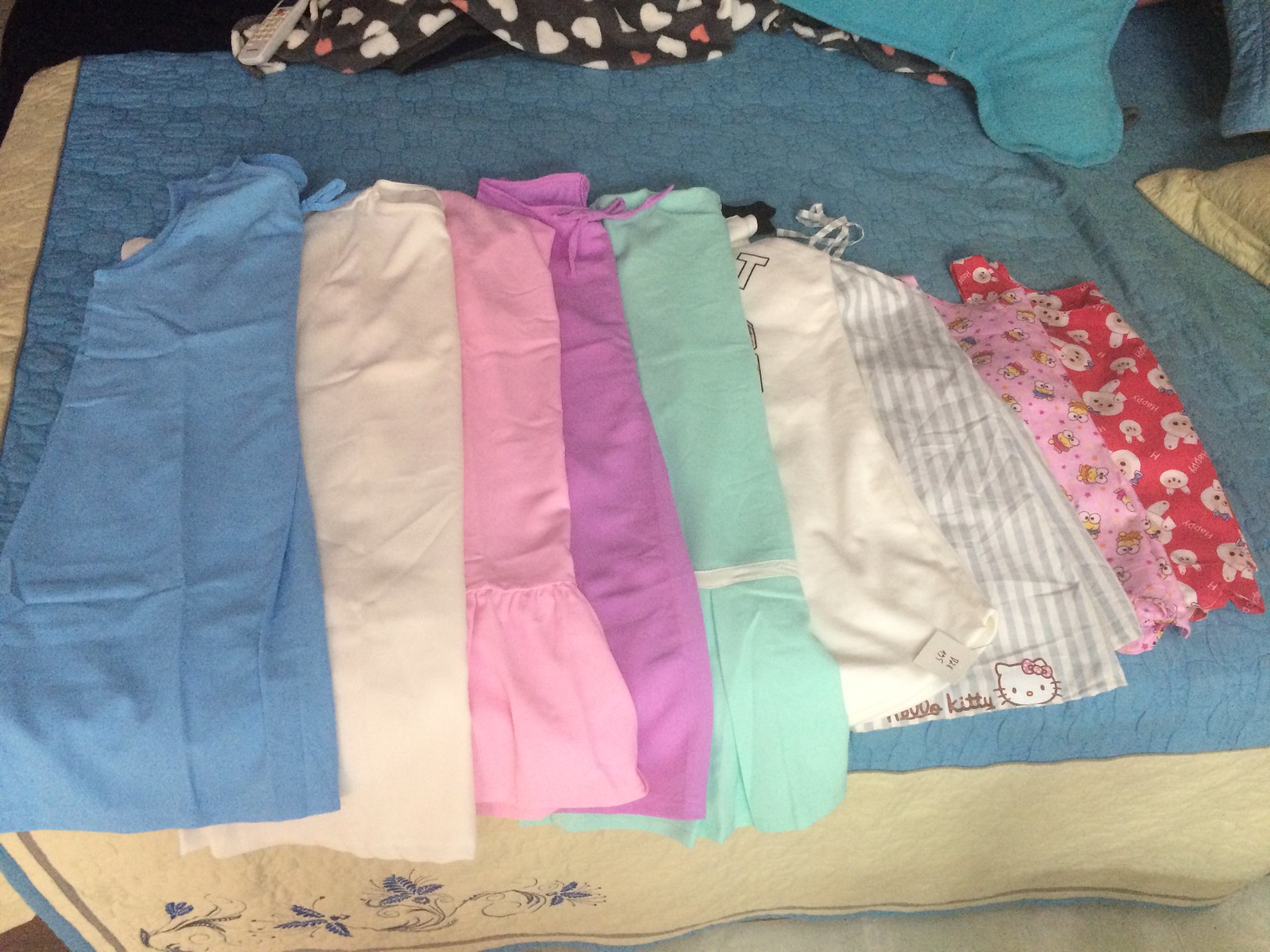This photograph depicts an assortment of children's clothing meticulously laid out in a neat row on a bed, each piece slightly overlapping the next. The bed, adorned with a blue and white quilt featuring butterfly patterns, adds an inviting, homey touch to the scene. Starting from the left, the clothes appear to be various aprons and possibly dresses or skirts, identifiable by their string ties. The first piece is a blue item, followed by a succession of colorful attire: a pink apron, a purplish-pink one, a teal-colored one, and a white piece. Notably, a white apron with gray stripes displays a Hello Kitty logo near the bottom. Following these are a pink apron adorned with little cartoon characters and a red piece featuring cartoon llamas or bunnies. The overall impression suggests a curated collection of children's clothing, possibly prepared for an online listing or an upcoming trip.